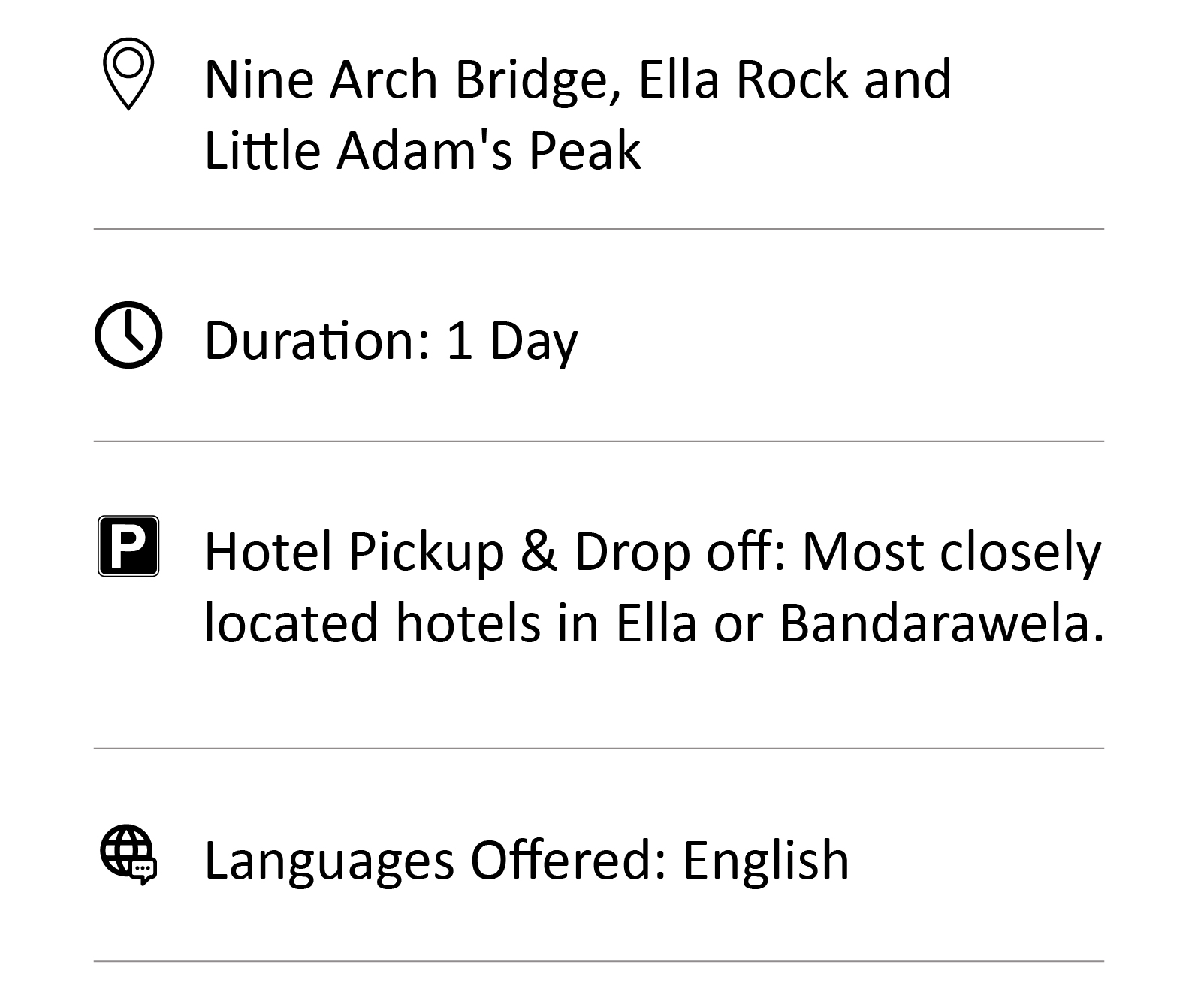An informative image presents details about a one-day tour covering some of Sri Lanka's most scenic attractions: the Nine Arch Bridge, Ella Rock, and Little Adam's Peak. The layout consists of four columns separated by black lines on a white background, with pertinent information displayed in black text.

1. **Tour Highlights**: 
   - **Nine Arch Bridge**: A renowned architectural marvel.
   - **Ella Rock**: A popular hiking destination with stunning views.
   - **Little Adam's Peak**: Known for its breathtaking panorama.

2. **Duration**: 
   - Indicated by a small clock icon, it specifies the tour lasts for one day.

3. **Hotel Pickup and Drop-off**:
   - Represented by a parking symbol, the service is available for hotels most closely located in Ella or Bandarwela (spelled B-A-N-D-A-R-A-W-E-L-A).

4. **Languages**:
   - Denoted by a globe and text bubble icon, the tour is offered in English. 

The overall design is clean and minimalist, ensuring the information is easily readable and accessible.